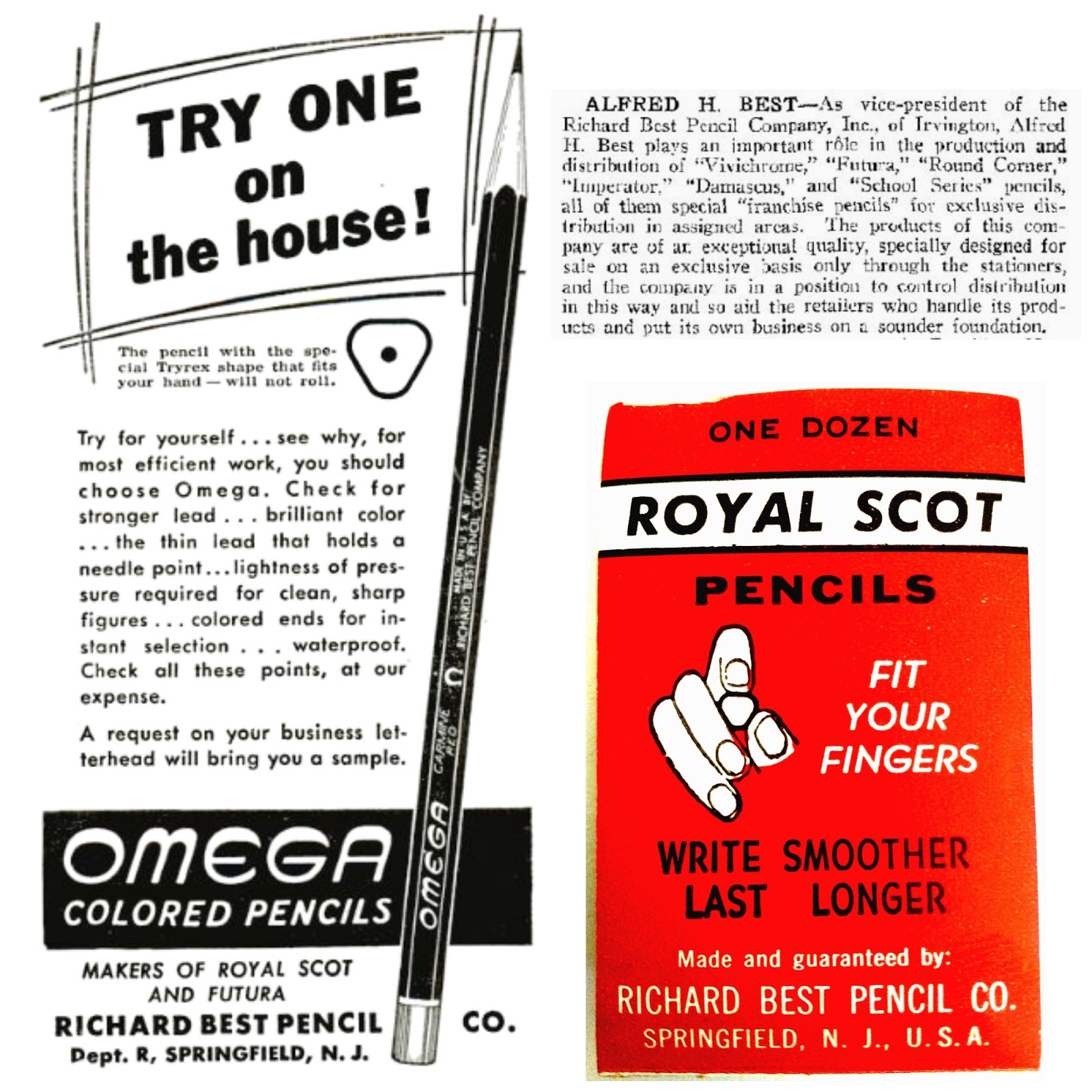This is a detailed magazine advertisement for Omega Colored Pencils by the Richard Best Pencil Company, featuring a striking mix of black, white, and red elements. The focal point is a bold red graphic announcing "One dozen Royal Scott pencils, fit your fingers, write smoother, last longer." It emphasizes the company's commitment to quality, stating, "Made and guaranteed by Richard Best Pencil Company, Springfield, New Jersey." On the left side, a banner highlights, "Try one on the house," promoting the unique Tyrex shape of the Omega pencils which fit comfortably in the hand. Detailed promotional text encourages readers to "Check for stronger lead, brilliant color, the thin lead that holds a needle point, and lightness of pressure required for clean, sharp figures." Additionally, it touts features like colored ends for easy selection and the pencils' waterproof quality. An image of a hand holding one of these pencils adds visual emphasis. The advertisement also mentions the involvement of Alfred H. Best as vice president, responsible for special franchise pencils, thus reinforcing the credibility and expertise behind the product.